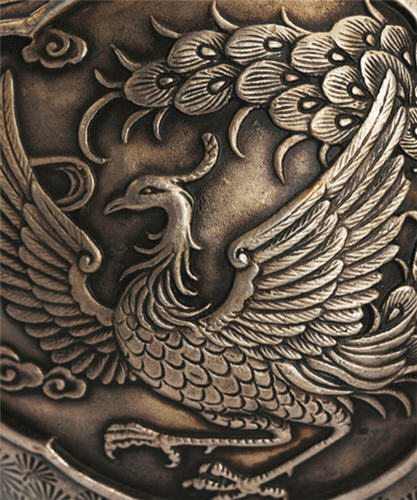The photograph captures a detailed image of a phoenix intricately designed on what appears to be a bronze or metallic surface, possibly a piece of jewelry or ornate pottery. The phoenix stands upright, with its wings extended elegantly to the sides, each feather meticulously rendered. Its long, slender neck is adorned with wiry feathers that cascade into more simplistic U-shaped feathers on its chest. Atop its head, a single feather curls upwards in an arch. The bird's bent legs end in sharp claws, adding to its majestic presence. The background includes additional scroll-like designs and possibly another wing or feathered element from a different bird, although this part remains ambiguous but does not detract from the main focus – the phoenix. The overall color scheme is a bronzy-silver with darkened edges, giving it an ancient, artistic feel.